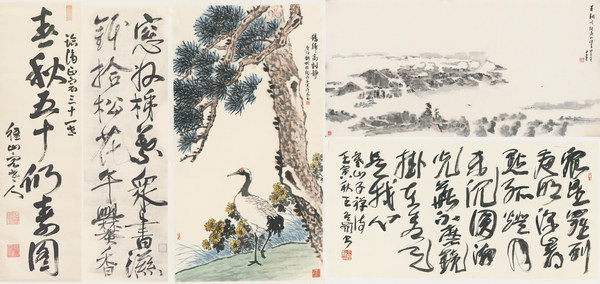This detailed watercolor illustration, in landscape layout, is broken down into five distinct segments composed of vertical and horizontal rectangles. The left side contains three vertical panels featuring Asian calligraphy—likely Japanese or Chinese—with intricate black ink lettering and occasional red accents on a cream background. The middle vertical panel showcases a detailed, color illustration of a pine tree with a brown trunk and green foliage, accompanied by a black and white crane with a splash of red on its head, standing amid green grass and yellow flowers. The right side features two horizontal panels stacked on top of each other: the upper panel displays a scenic black and gray landscape painting depicting mountainous terrain, land, and trees against a cream background, while the lower panel continues the theme of Asian text with black characters on a cream backdrop.